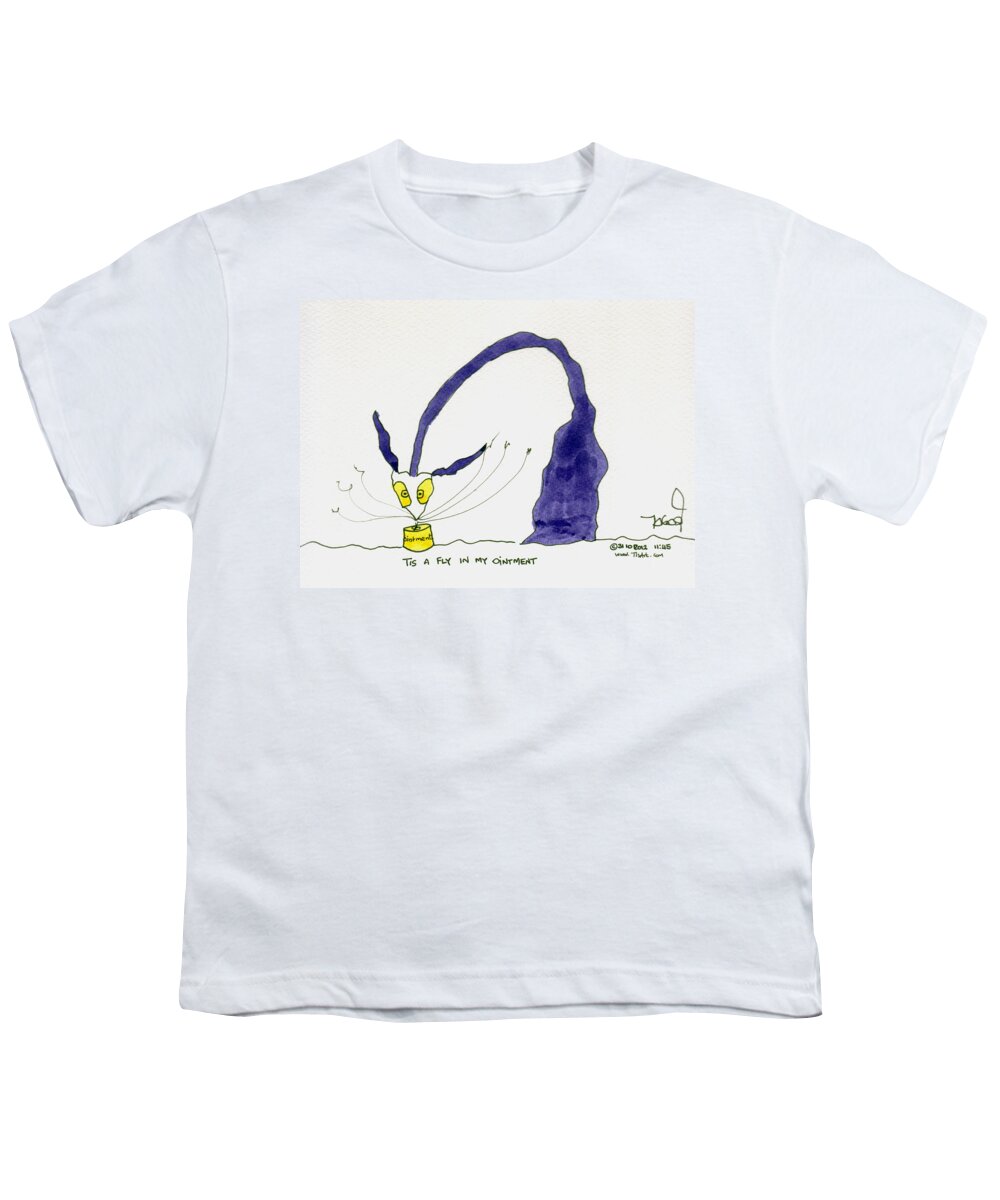The image features a white cotton crewneck t-shirt displayed against a white background, giving it a floating appearance. The t-shirt, which is slightly wrinkled and short-sleeved, displays the "Fly in the Ointment" design on the front. Centered just below the neckline is a beige rectangular section that frames the graphic. The design portrays a whimsical, long-necked, purple creature with a triangular white head, large yellow eyes, and elongated ears bending towards a circular yellow tin of ointment. This fantastical figure has a dark blue neck that narrows at the top and curves to the left. Black lines seem to depict the creature's arms, with three on each side, and a black squiggly line represents the ground beneath the illustration. Several flies are shown flying out of the ointment tin, with three on each side. Below the graphic is black text that reads, "Tis a fly in my ointment," accompanied by a barely visible artist signature to the right.